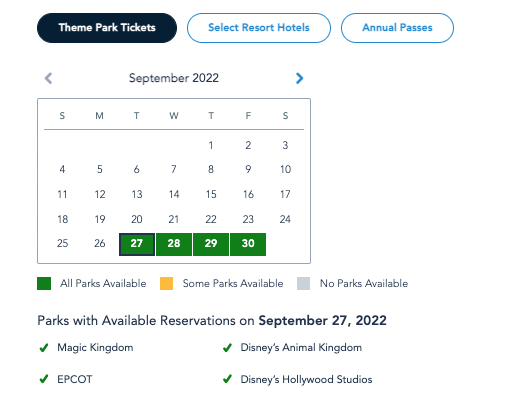The image appears to be a screenshot from a Disney reservation system. At the top, there are three tabs: "Theme Park Tickets," "Select Resort Hotels," and "Annual Passes." The "Theme Park Tickets" tab is highlighted in dark blue, while the other two tabs are outlined in blue with a white background. 

The calendar is set to September 2022, with specific dates highlighted: the 27th, 28th, 29th, and 30th, representing Tuesday through Friday, respectively. These dates are marked in green, indicating that all parks are available. A legend explains the color coding: green means all parks are available, yellow signifies some parks are available, and gray indicates no parks are available.

Below the calendar, there is a list of parks with available reservations for September 27th, 2022. Each park listed has a green checkmark next to it, indicating availability. The parks listed include:
- Magic Kingdom
- Disney's Animal Kingdom
- Epcot
- Disney's Hollywood Studios

Additional navigation options, such as forward and backward arrows, are present near the calendar, presumably to switch between months. The "Theme Park Tickets" tab is styled in a navy blue to black gradient with white text. The image does not show any other parts of the web page or app beyond this reservation interface.